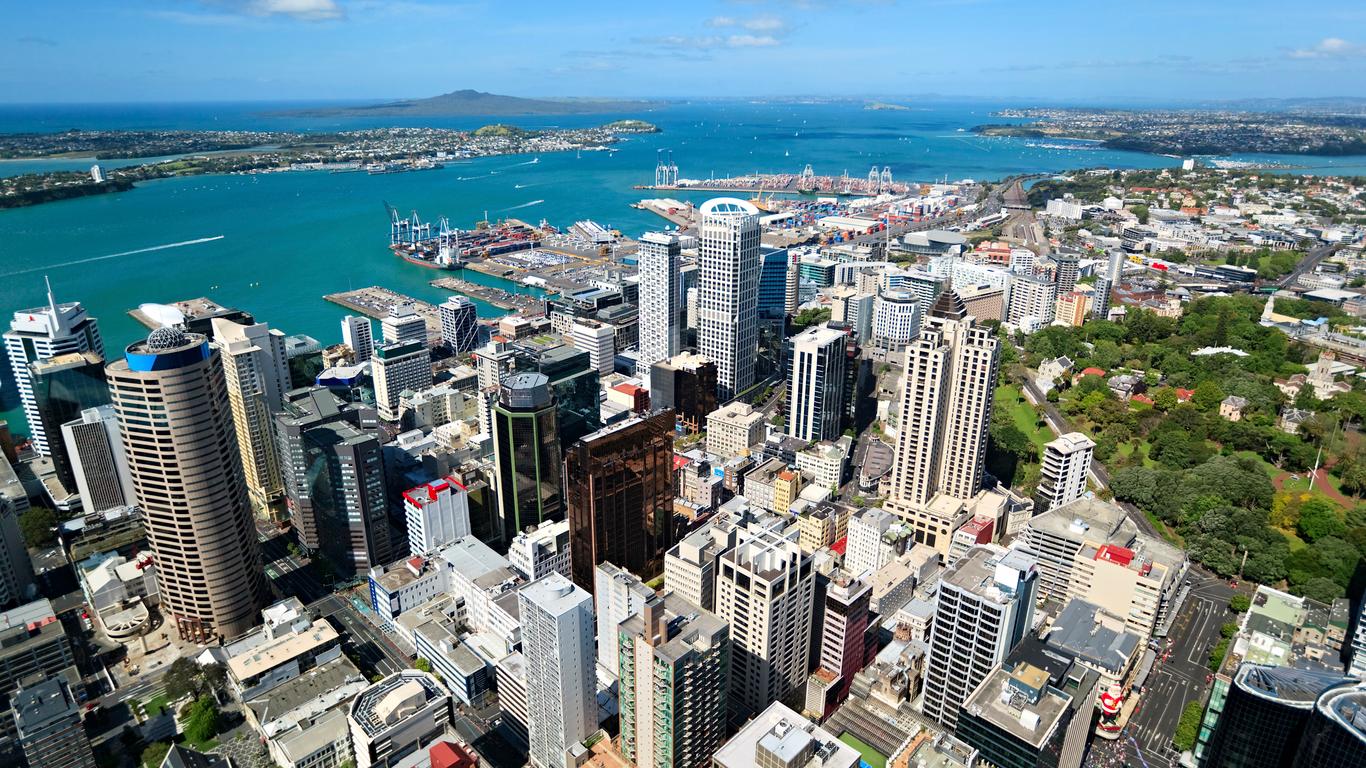Aerial photograph showcasing a bustling modern cityscape, comprising numerous tall skyscrapers and high-rise buildings in various shades of gray, white, black, and silver. Several of these structures are sheathed in glass, while others appear to be constructed from concrete. Prominently, a triangular prism-shaped building with a brown exterior stands on the left, contrasted by a striking, dark glass building in the center.

The city's layout reveals a dense urban grid interspersed with streets, and a mix of architectural styles and shapes. There is a unique cylindrical building with green vertical lines, as well as a sprawling area of low-rise buildings towards the upper right, complemented by green spaces filled with trees in diverse shades.

In the background, a large body of water, likely a harbor or bay, prominently features, flanked by two landmasses resembling peninsulas pointing towards each other. The water is a vibrant blue, dotted with piers and boats. On the left, multiple piers jut into the water, some equipped with mechanical cranes. The far horizon showcases a low mountain or island, with subtle mountain ranges extending into the distance.

Above this urban and natural tableau, a mostly clear blue sky with scattered white clouds further enhances the scene. This photograph effectively captures the dynamic and multifaceted essence of a major coastal city.